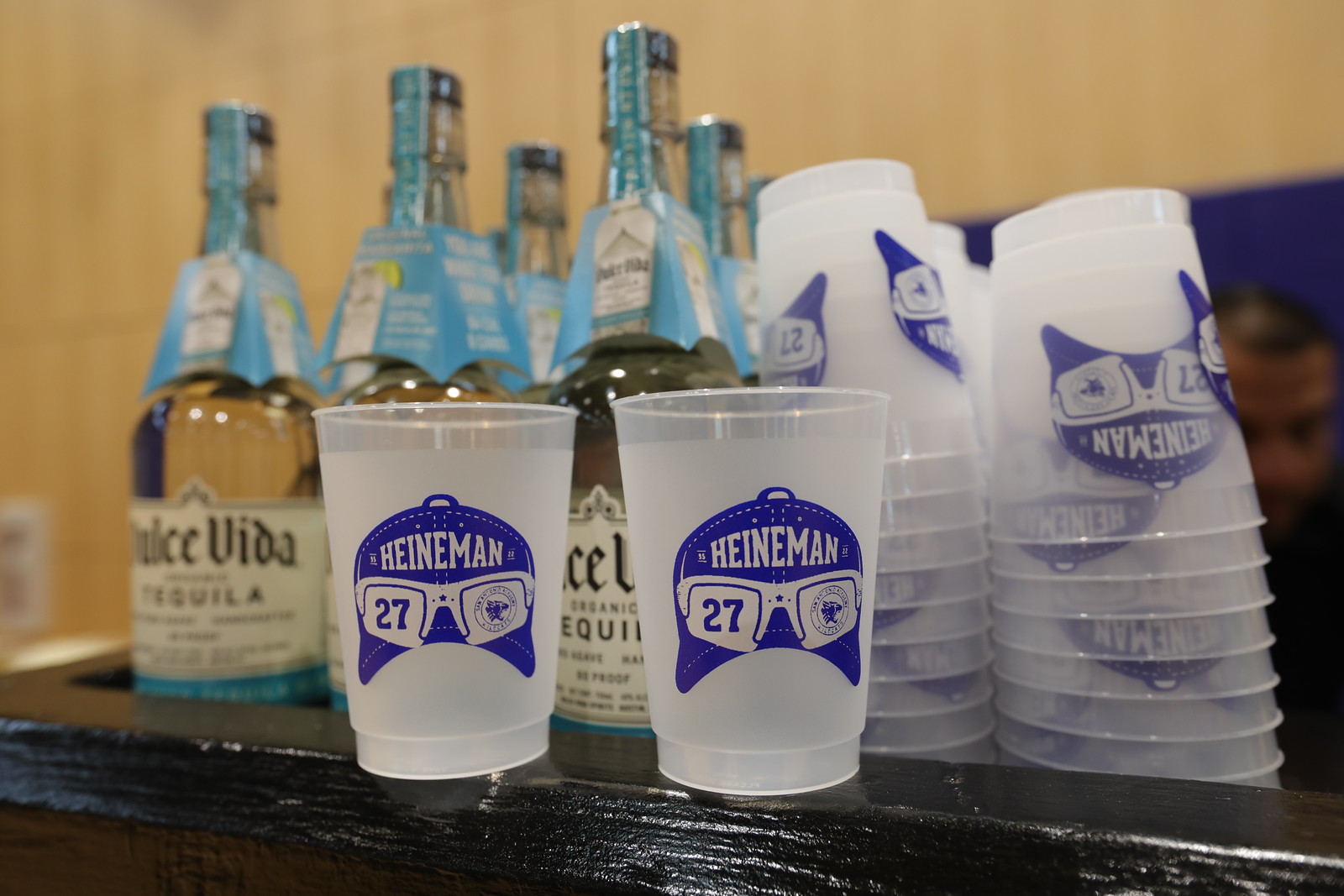The photograph, taken indoors, showcases a bar area prominently featuring plastic cups and bottles of tequila. Two semi-transparent plastic cups, adorned with a blue baseball cap with sunglasses and the brand name "Heinemann," are placed right side up on a wooden bar ledge. The cap graphics include the number 27 on the left lens of the sunglasses and another symbol on the right. Behind these cups, several more plastic cups are stacked upside down in multiple piles. To the left of these cup stacks, there are rows of "Dolce Vita Tequila" bottles, each featuring blue cardboard tops. A blurry image of a man, possibly a bartender, is visible in the background to the right, adding a human element to the scene. The background also includes a tan-colored wall with a light socket visible on the left edge.